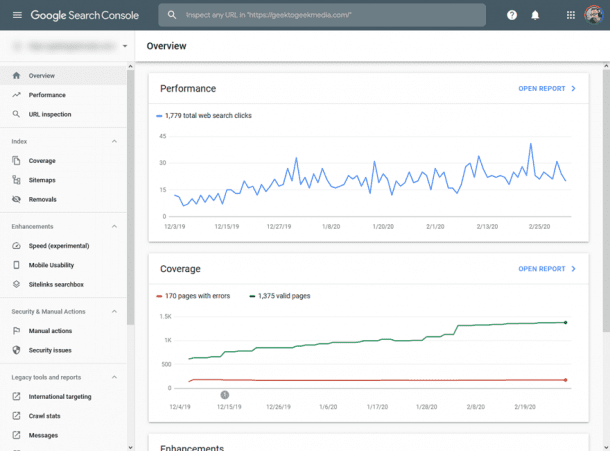The image showcases the interface of the Google Search Console. At the top, there is a wide, dark gray banner with light gray lettering that reads "Google Search Console." To the left of this text are three horizontal lines. Centrally located within the dark gray banner is a lighter gray search bar, accompanied by a magnifying glass icon on its left, symbolizing a search function. 

To the right of the gray banner lies a white circle containing a question mark, likely indicating a help or information feature. Adjacent to this are a white notification bell and an icon featuring three vertical dots, symbolizing additional settings or options. Further to the right, there is a small circular user profile image.

Beneath the gray banner, the background is predominantly white. On the left side of the page, there is a vertical navigation menu containing about five groups of three categories each. In the center of the main content area are two charts. The upper chart, labeled "Performance," features blue line graphs, while the lower chart, titled "Coverage," displays green and red lines indicating different data metrics.